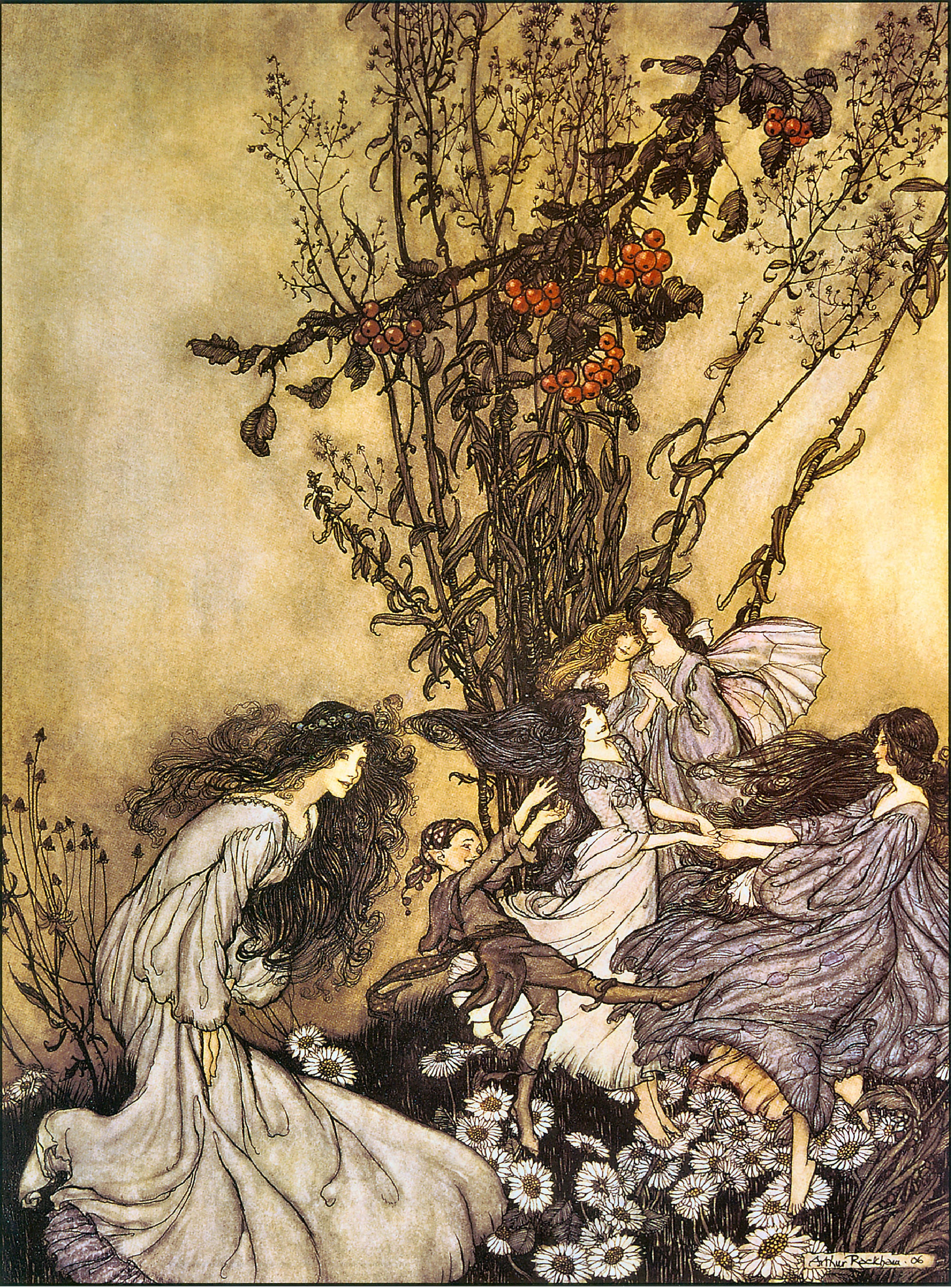An intricate illustration from an 1800s-era book showcases a whimsical scene rendered in pen and ink with watercolor accents, set against a tan and yellow backdrop. To the left stands a young woman with waist-length, curly flowing hair, adorned with a flower headband. She is dressed in a billowing white gown with long sleeves that catch the wind. On the right, three female figures resembling fairies, dressed in gray dresses with matching wings, hold the hands of a fourth woman. This central figure wears an elaborate, low-cut white gown from the same period with her hair elegantly pinned up. In the middle of the scene, between these groups, dances a small sprite-like character dressed in a jagged-edged dark skirt over tights. The background reveals detailed ink and watercolor sketches of plant stalks and vines adorned with red berries, reminiscent of holly. The scene is set in a nature field abundant with daisies and mushrooms, under a sky bathed in golden hues. The bottom right corner shows an indistinct signature of the artist.